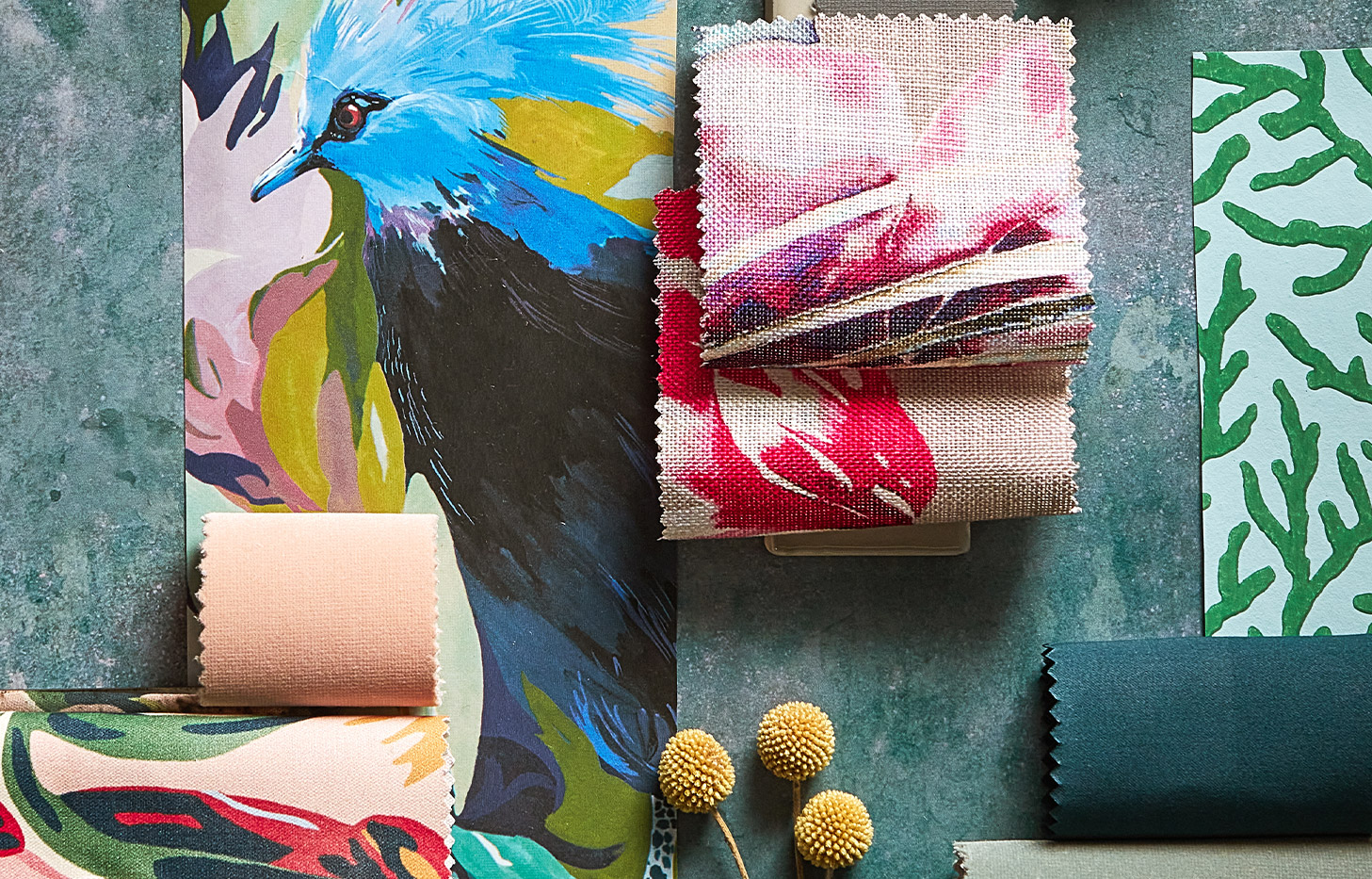This color photograph showcases an artistic work-in-progress setup on a bluish-green, concrete-style table. The table is adorned with a mixture of vibrant fabric and wallpaper swatches, evoking a tropical and abstract theme. On the left side, prominently displayed, is an incomplete yet striking painting of a blue bird with ruffled head feathers and a crest. Adjacent to the bird painting is another artwork featuring a bird with a black body and blue near its legs, highlighting the varied artistic experiments taking place.

Centrally, the table features an assortment of fabric swatches with serrated edges, including brightly colored fabrics that boast tropical floral designs in reds, blues, and pinks. There's also a piece with a white background displaying green coral-like patterns. In addition to these, laid out are folded fabrics embellished with painted designs, adding to the creative chaos.

Towards the bottom left, a vivid patch of wallpaper showcases a fusion of peaches, reds, blues, and greens, harmonizing with the overall tropical aesthetic. Amidst these elements are three small, dried yellow pom-pom-like flowers on sticks, adding a touch of whimsical texture to the tableau. The entire arrangement gives an impression of an artist's lively and colorful workspace, with both completed and in-progress pieces hinting at the creative process behind the scenes.